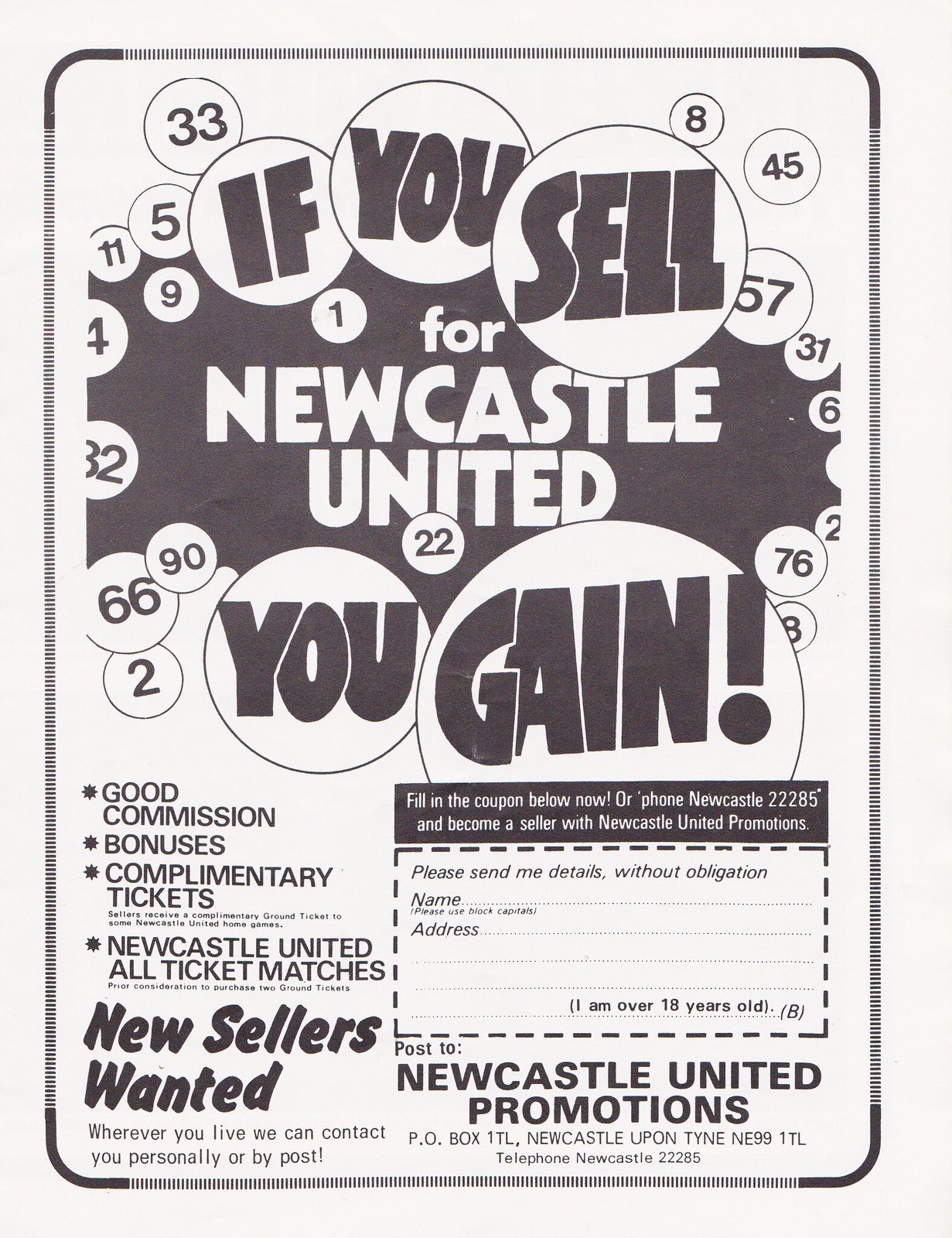This is a black and white advertisement, likely from the 1940s or 1950s, appearing in a newspaper or magazine. The upper section features a black oval surrounded by white circles containing various numbers, reminiscent of bingo balls. The text within these circles reads, "If you sell," and, "You gain," with the phrase "for Newcastle United" displayed prominently in white text against the black oval.

Below this attention-grabbing header, the advertisement lists enticing incentives such as good commissions, bonuses, complimentary tickets, and access to all-ticket matches for Newcastle United's home games. It emphasizes the desirability of becoming a seller for Newcastle United Promotions by stating, "New Sellers Wanted. Wherever you live, we can contact you personally or by post."

The bottom right section contains a coupon for prospective sellers to fill out with their name and address, clearly intended for individuals over 18 years old. It encourages immediate action with the prompt, "Fill in the coupon below or phone Newcastle 22285 and become a seller of Newcastle United promotions." The advertisement closes with the contact information for Newcastle United Promotions, P.O. Box 1TL, Newcastle upon Tyne, ND99 1TL, and the telephone number: Newcastle 22285.